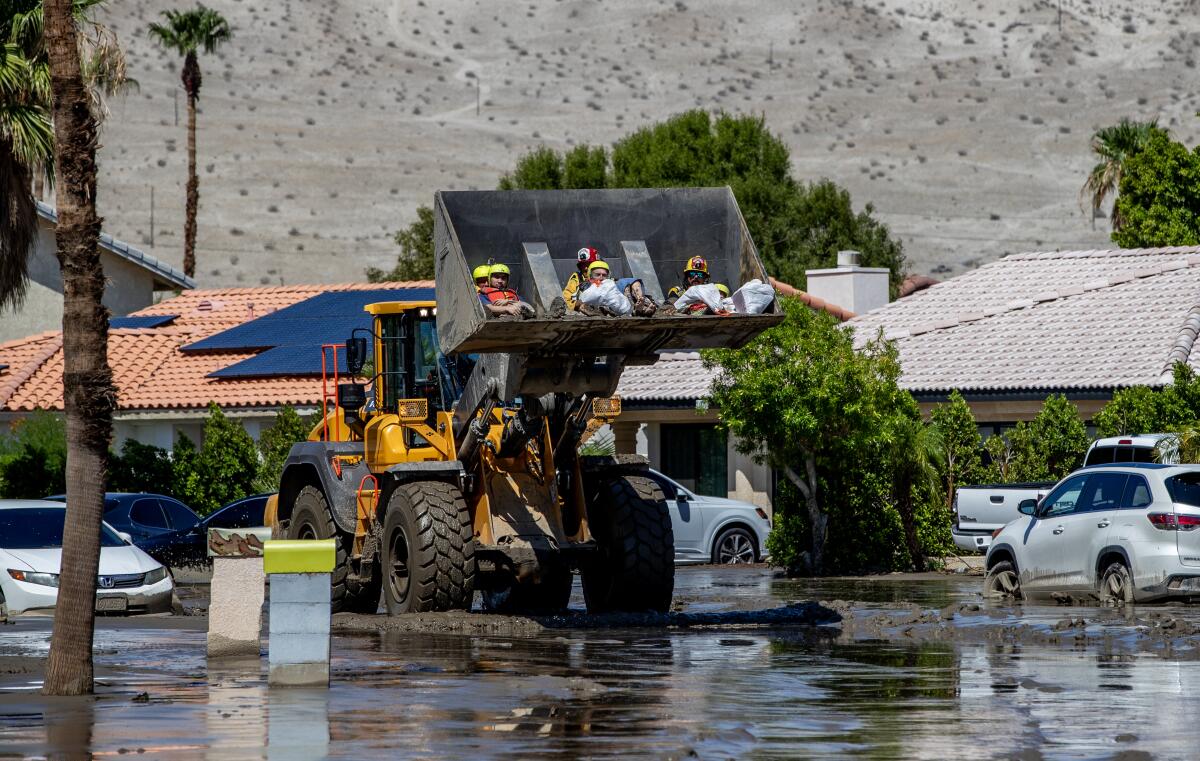In the midst of a sprawling desert landscape with dry, barren surroundings dotted with sparse greenery, a striking scene unfolds in a flooded neighborhood. The area is inundated with water and mud, affecting several desert-style houses with tile roofs, one of which is equipped with solar panels. Towering, slender palm trees stand amidst the chaos, their green fronds providing a stark contrast to the muddy waters below. 

Central to the scene is a yellow front-end loader, typically used for shoveling materials like dirt and gravel, but now repurposed for an urgent rescue operation. The shovel attachment, raised above the muddy ground, contains several helmeted individuals. It is unclear whether they are rescue or cleanup workers, but their presence underscores the severity of the situation. The loader navigates through the mud, likely either ferrying these men to safety or transporting them to assist in the rescue of others affected by the apparent flash flood.